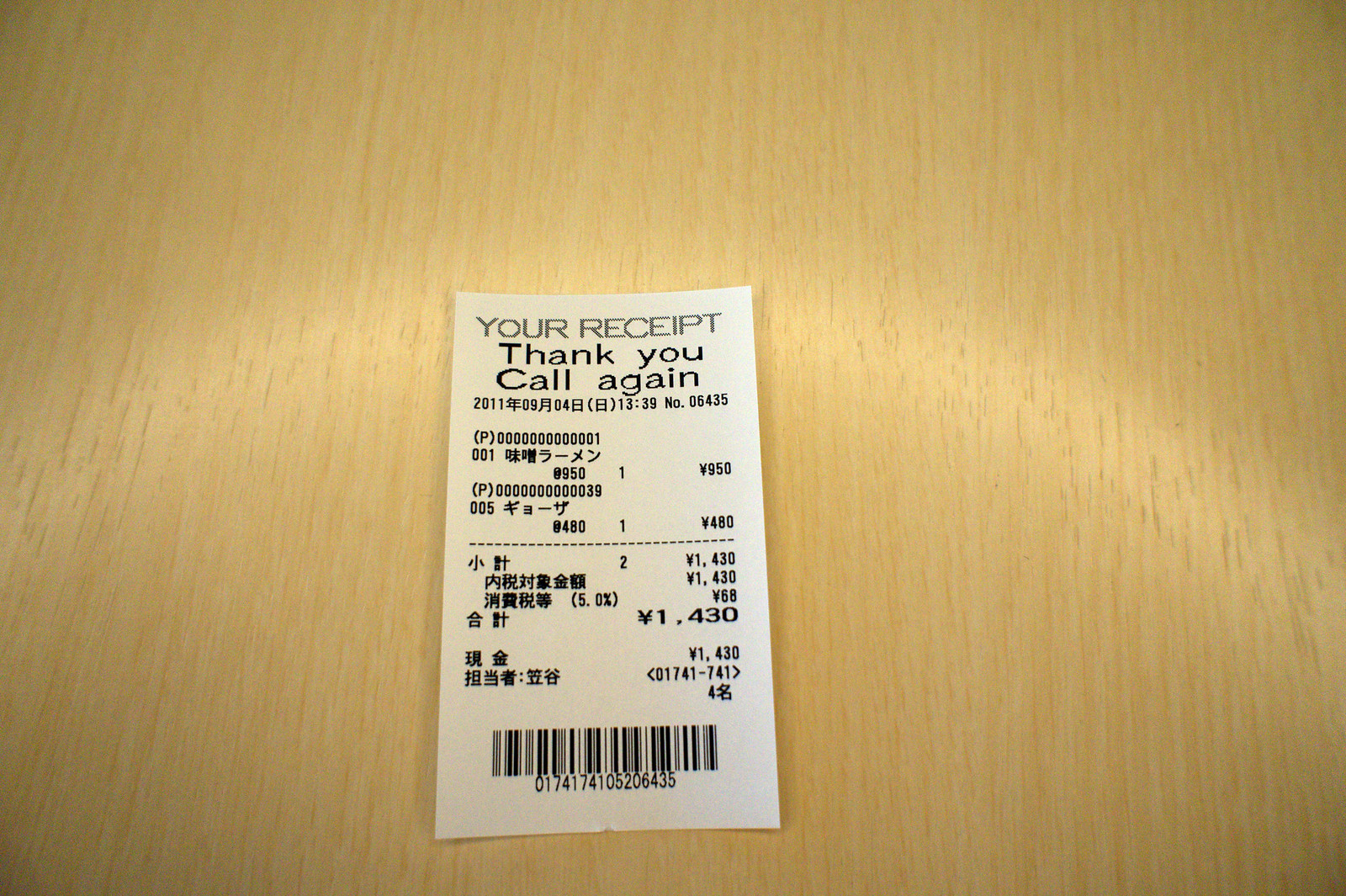A rectangular receipt lies on a beige wooden surface, predominantly white with most of the text in black. At the top, the phrase "YOUR RECEIPT" is prominently displayed in uppercase letters, rendered in a dark gray color. Directly below, the receipt extends a courteous note: "Thank you, thank you, call again." 

In the subsequent section, a sequence of characters including numerals and Asian script reads "2011 八重洲 09 八重洲 04 八重洲," followed by additional text in Asian script that is partially obscured. Adjacent to this, the letter "P" enclosed in parentheses is visible along with a series of zeros and a one.

Further down, the receipt displays "001 八重洲 0950" and continues a similar pattern, presenting "0480" beneath another set of Asian characters. On the left side at the bottom of the receipt, more Asian characters are noted, juxtaposed by the number "1,430" on the right side. The receipt concludes with a barcode at the very bottom.